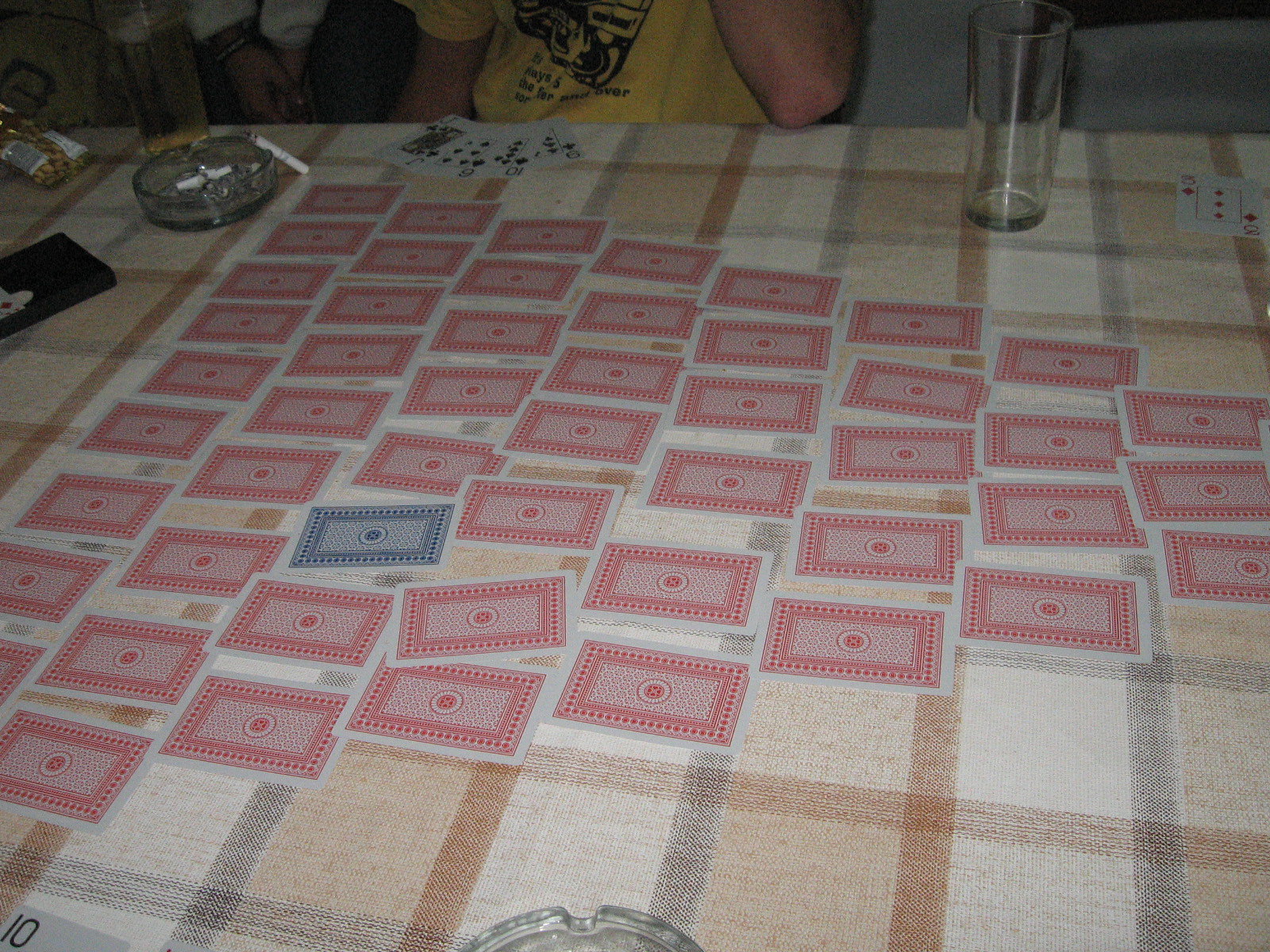In this detailed image, a spirited card game is taking place on a table adorned with a tan, brown, and black plaid cloth. At the bottom center, a clear glass ashtray can be seen, holding one white cigarette and another leaning against it on the top left. A glass cup is positioned on the top right side of the table. Dominating the scene is a tower of cards, with predominantly red backs and a single blue card, showcasing the players' creativity. An aluminum card with a metallic sheen lies in the bottom left.

Across the table, a spread of five diamond cards and additional face-up cards are present, hinting at an ongoing game. A person in a yellow shirt with black writing is engaged in the game. On the left side of the table, a black box and a bag of snacks rest in the top left corner. The hands of another participant, wearing a white shirt or sweater, are visible on the top left, along with the edge of a chair or its arm, adding to the cozy, intimate setting of this friendly gathering.